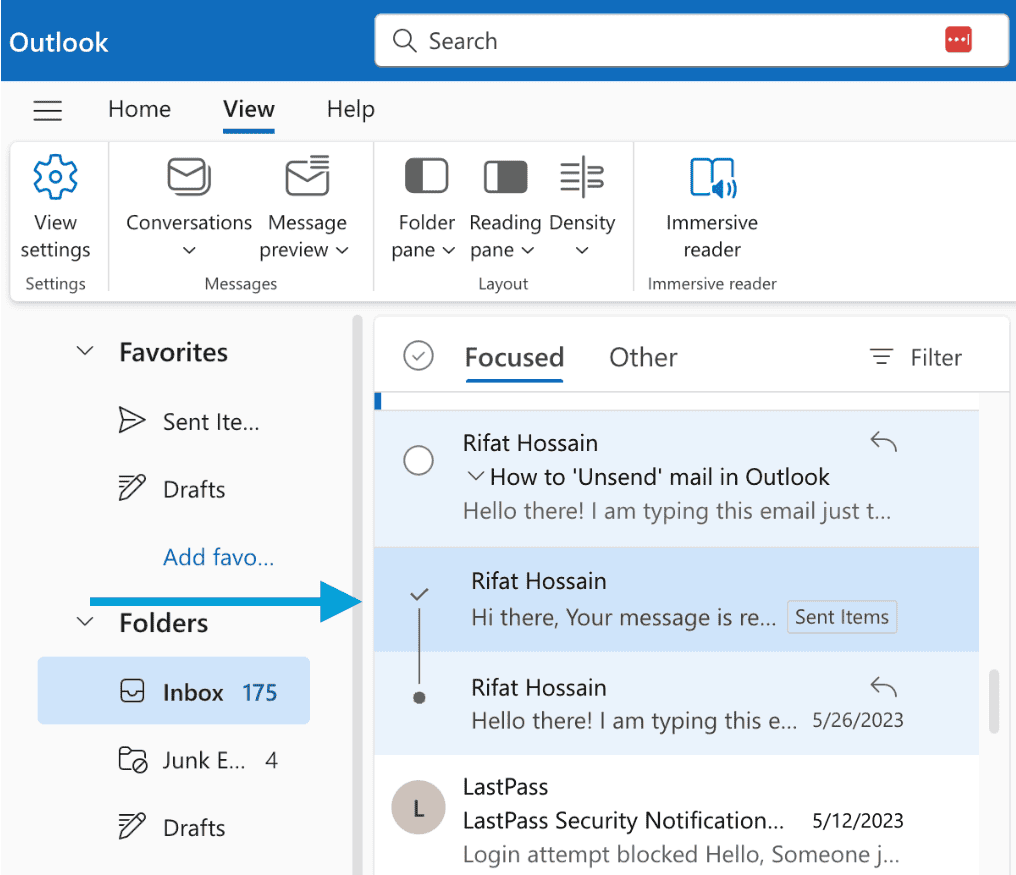The image depicts the Outlook email interface. At the top, there's a dark blue bar labeled "Outlook," accompanied by a search bar with a magnifying glass icon. Beneath this, a toolbar with the options "Home," "View," and "Help" is displayed. Following this toolbar, options like "View Settings," "Conversation," "Message Preview," "Messages," "Folder Pane," "Reading Pane," "Layout," "Density," and "Immersive Reader" are listed.

On the left sidebar, numerous folders and categories are visible, including "Favorites," "Sent Items," "Drafts," "Add Favorites," "Folders," "Inbox (175)," "Junk Emails (4)," and "Drafts." Adjacent to this sidebar, a section featuring a white background at the top presents a circle with a checkmark, labeled "Focus," with a blue underline, and "Others" to its right. On the far right of this section, there's a "Filter" option represented by three horizontal lines.

Below the filter option, there's a light blue area with a white circle on the left. Inside this area, text in black reads: "Rifat Hossain, How to Unsend Mail in Outlook. Hello there, I'm typing this email."

This structured interface showcases various functionalities and navigational elements of Outlook, designed to streamline email management and enhance user productivity.